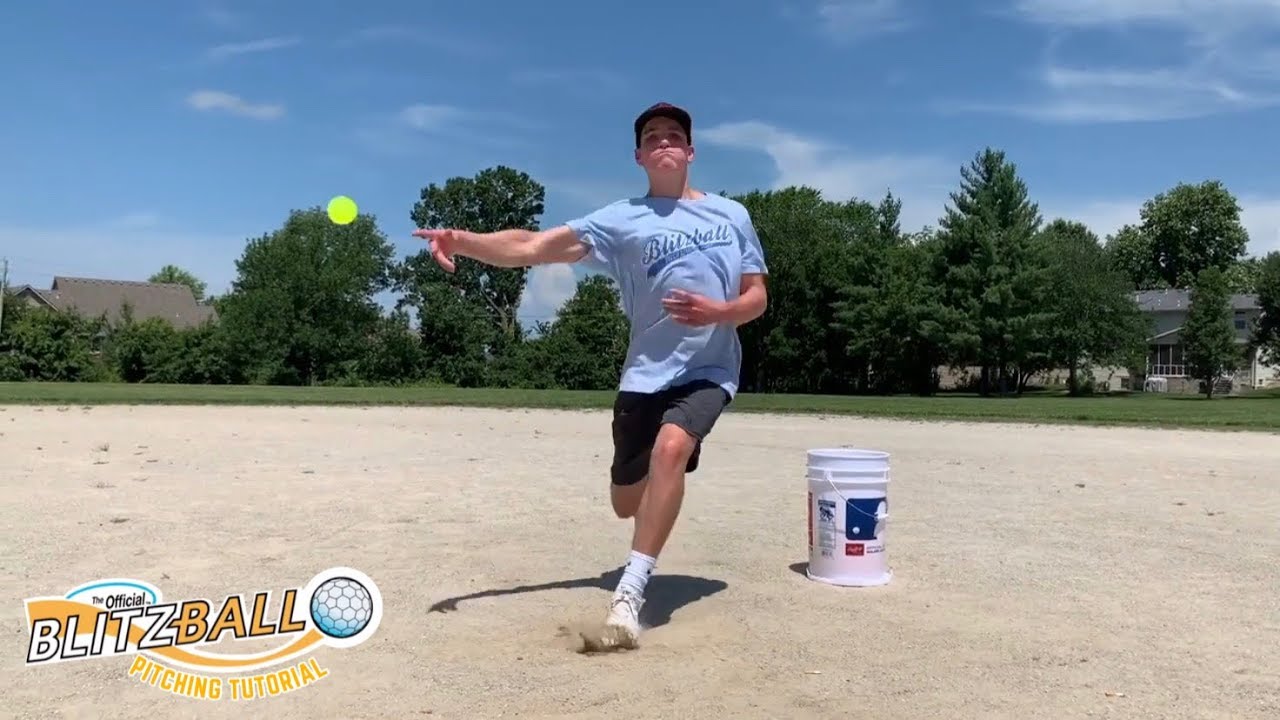In this rectangular picture, a teenage boy is captured in mid-pitch, seemingly in the midst of an intense and aggressive throw. He is fair-skinned and wears a dark cap, a short-sleeved blue shirt emblazoned with the word "Blitzball" in blue, black shorts, white socks, and white shoes. The boy is throwing a yellow ball that lacks discernible lines, characteristic of the unique Blitzball. To his right sits a white bucket, presumably filled with more balls, sporting a red, white, and blue logo. 

The backdrop reveals a serene suburban setting, with a bright blue sky punctuated by a few clouds. In the distance, two houses framed by a copse of trees are visible, creating a picturesque residential vibe. The scene appears to take place in a sandy, grass-edged area, adding to the casual outdoor atmosphere.

A prominent logo in the bottom left corner reads "The Official Blitzball Pitching Tutorial." This logo features an orange swoosh running through the text "Blitzball," complemented by an image of a ball that resembles a shrunk-down, hexagon-covered version of a golf or soccer ball, highlighting the unique design of the Blitzball.